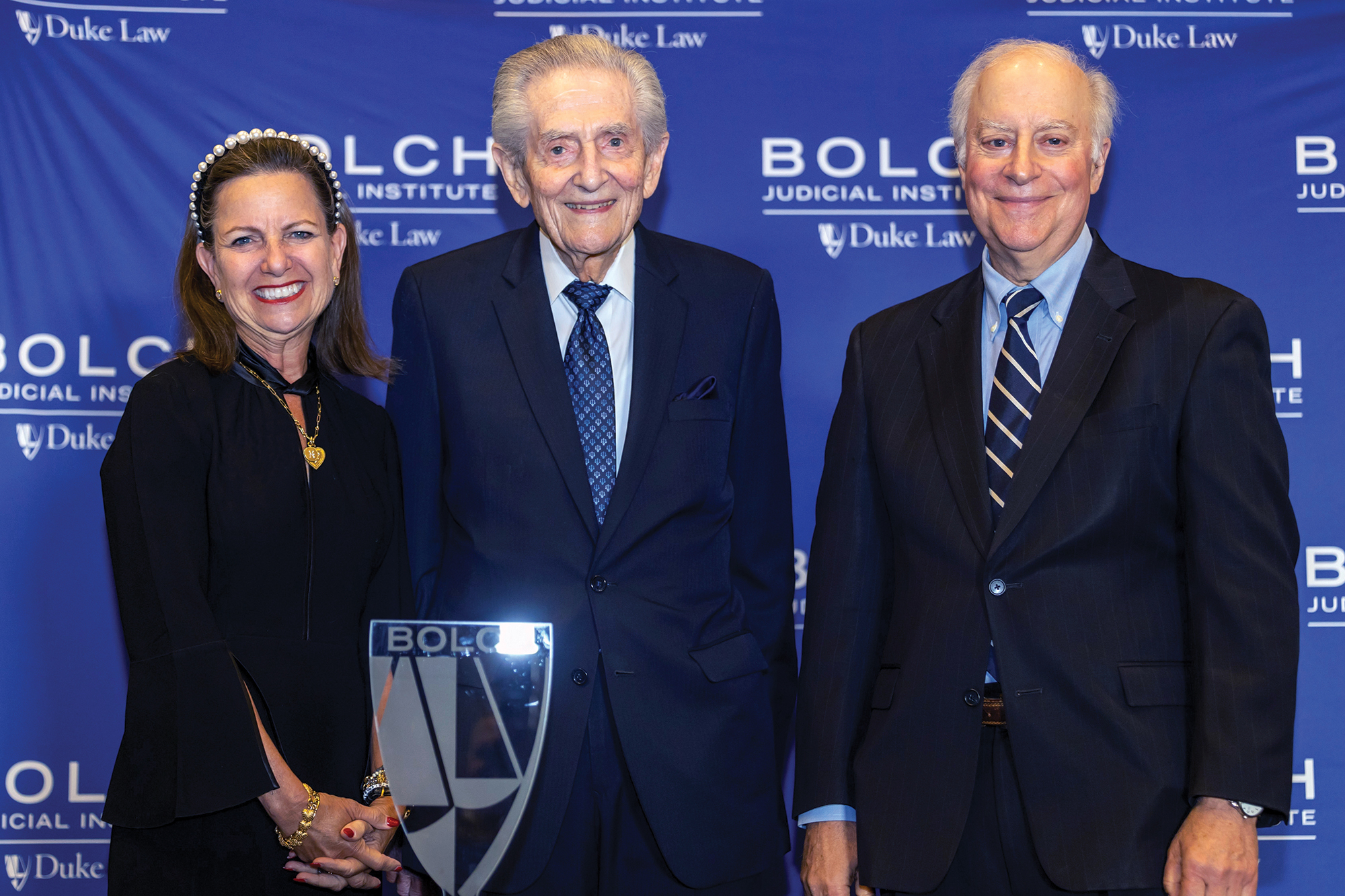In this color photograph, three individuals are standing in front of a purpley-blue backdrop decorated with white lettering that reads "Bolch Judicial Institute" and "Duke Law," accompanied by the Duke Law cross logo. The trio appears to be receiving an award or some form of recognition. On the left is a light-skinned woman with shoulder-length black hair adorned with a pearl crown or headband. She is dressed in a formal black top and dress, wearing a gold heart-shaped pendant on a silver necklace around her neck. She smiles broadly, displaying her top teeth, and has her hands folded in front of her. 

Next to her stands an elderly, light-skinned man, probably in his 80s, dressed in a blue suit with a blue patterned tie and a white shirt. To the right of him is another light-skinned man, who, although younger, is bald with gray hair on the sides. He wears a black suit with a blue button-down collared shirt and a blue tie featuring horizontal diagonal stripes. In front of the group is a lucite or glass trophy with the inscription "B-O-L-C-H" and an engraved logo, indicating it is an award. The atmosphere is positive, with all three individuals smiling and looking happy, posing for the photograph.